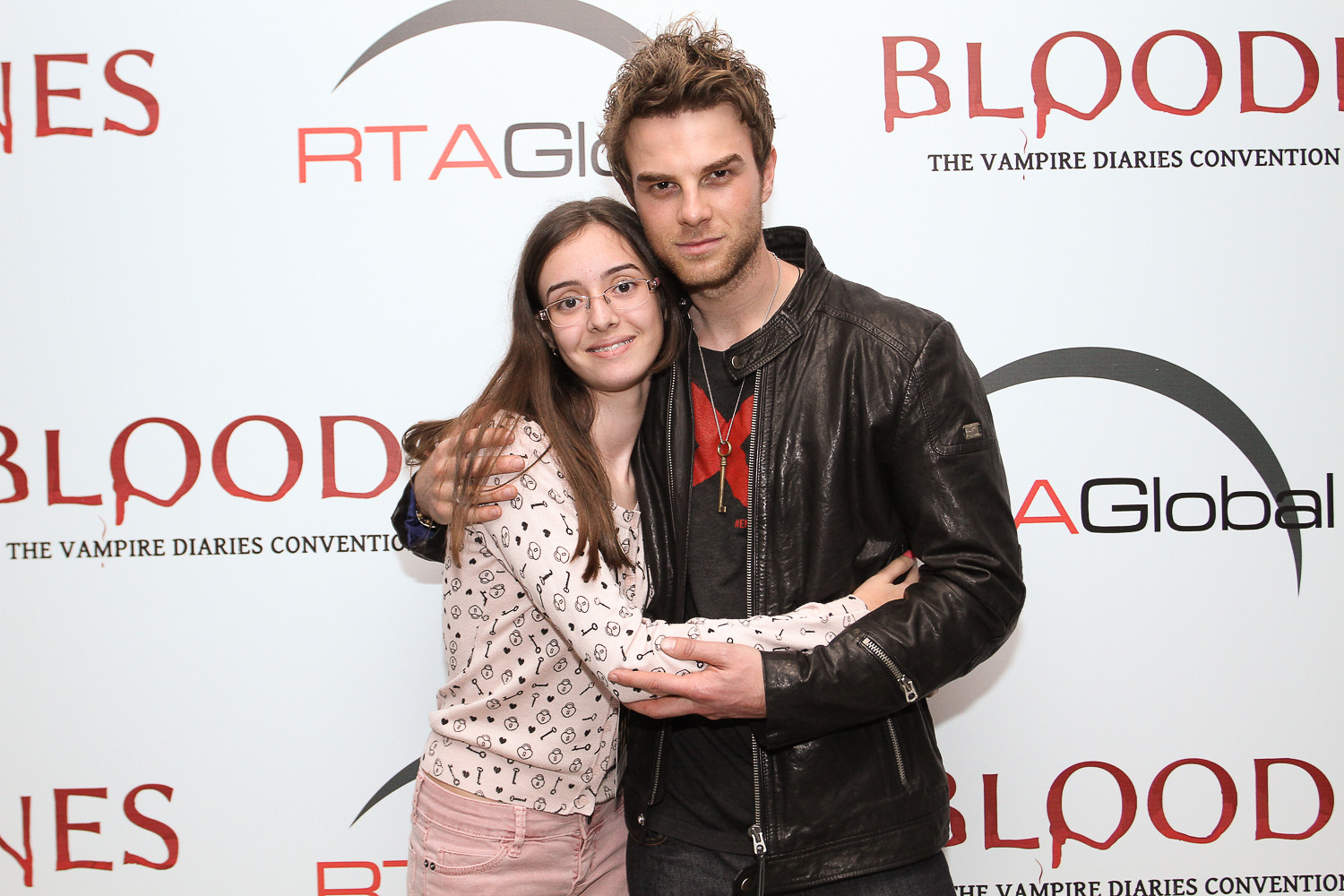In this indoor setting, a man and a woman are posing for a photograph at what appears to be a convention centered around the TV show "The Vampire Diaries." They are positioned directly in the center of the image, with a background featuring a white curtain patterned with red and black text that reads "Blood, The Vampire Diaries Convention, RTA Global." The man, standing on the right, is dressed in a black leather jacket over a black t-shirt, accessorized with a necklace that has a large key pendant. He has short, curly, dirty blonde hair and wears a serious expression. The woman, on the left, is leaning into the man, smiling warmly at the camera. She has long, straight brown hair and is wearing eyeglasses, a beige sweater with key graphics, and pink denim pants. The camaraderie between the two suggests she might be a fan meeting the actor at this event. The color palette of the image includes shades of white, red, black, pink, and silver, and while the exact time of day is unclear, the image exudes the typical bustling atmosphere of a convention.